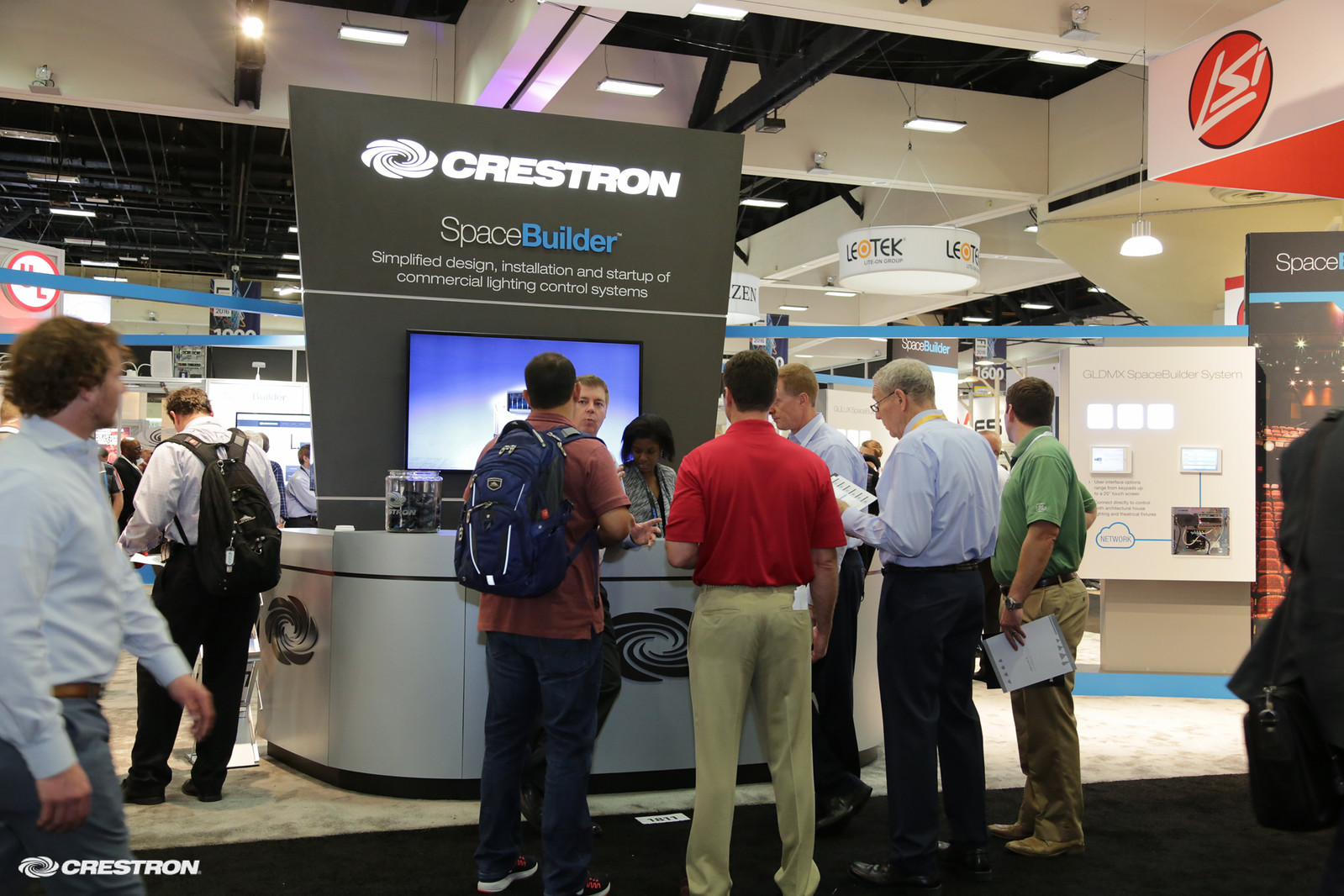The image captures a bustling scene in a large convention center, showcasing a prominent booth for Crestron, a company specializing in commercial lighting control systems. Front and center is a sleek white desk adorned with a black Whirlpool icon on its front and sides. Behind this desk, a tall gray sign illuminated in white lights features the Crestron logo and the text "SPACEBUILDER" with "SPACE" in gray and "BUILDER" in bold blue. Beneath this, it reads "Simplified design, installation, and startup of commercial lighting control systems." Two people are stationed behind the desk, engaging with a crowd of about six individuals, while additional attendees can be seen mingling around the booth area. To the left, a man with a large black backpack is noticeable, and to the right, there is a partial view of another person carrying a bag. The backdrop of the convention center reveals its unfinished ceiling with visible hanging lights, enhancing the industrial ambiance. Scattered throughout the space are other booths and signage, highlighting the conference setting dedicated to various businesses and technologies.